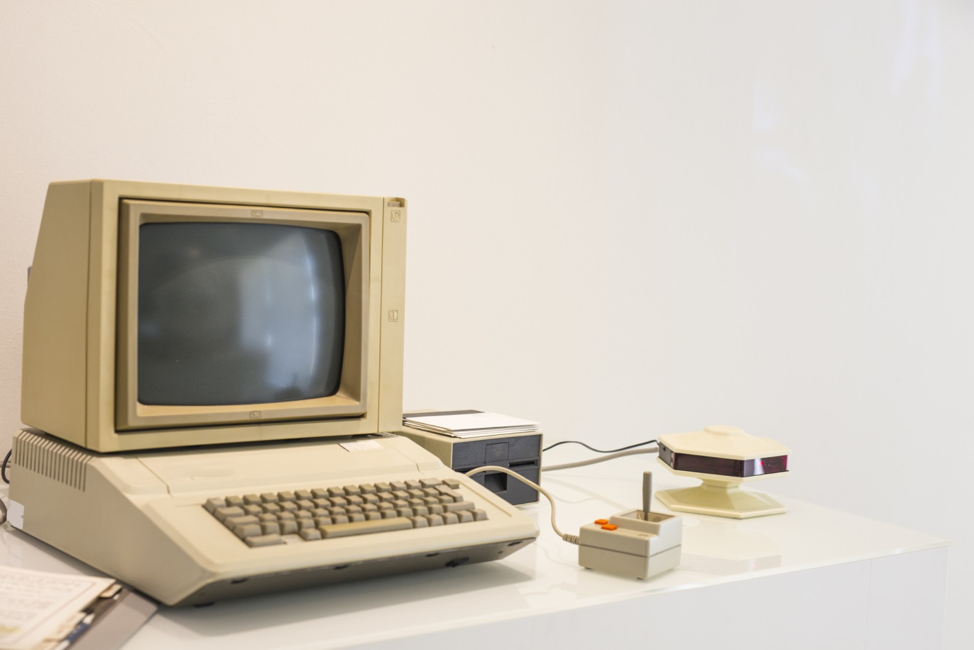The image is a color photograph in landscape orientation, showcasing a vintage computer setup prominently positioned on the left side of the frame. The computer rests on a white and red table, blending into the predominantly white background. The central component is an old-fashioned computer with a square, convex monitor housed in a light beige to brownish-beige plastic case, featuring a notably thick frame and back.

Below the monitor is a protruding, slanted keyboard section with raised beige keys on a light beige background. Extending from the keyboard's right side is a separate floppy disk drive with a dark gray front panel, alongside two additional attachments connected by wires. One notable attachment is a joystick, distinguished by its darker gray body and orange buttons.

Alongside the computer setup, various hexagonal-shaped objects and some papers can be seen scattered on the tabletop, adding to the scene's detailing. The detailed intricacies and arrangement of the computer and its peripherals create a vivid representation of early computing technology.